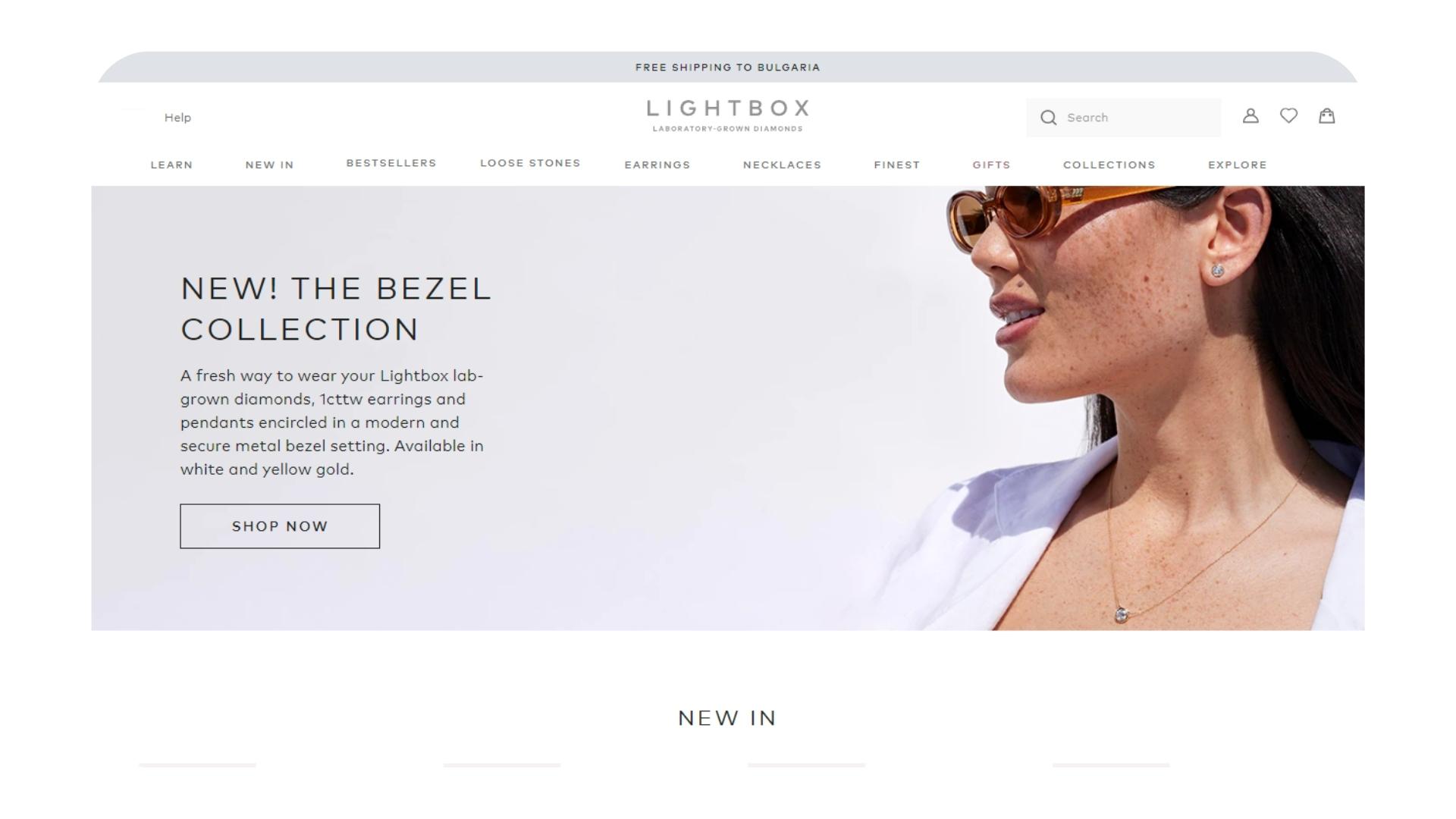This image depicts the upper section of a website, approximately two and a half times wider than it is tall. The entire background is a light gray, except for the white menu area. At the very top, above the menu, there is a gray strip with black text centered in all capital letters that reads: "Free Shipping to Bulgaria."

In the menu area, starting from the top left, there is the word "HELP" in black text. Centrally positioned, in larger gray text, it says "Lightbox" in uppercase, and underneath this in a very small font, it reads "Laboratory Grown Diamonds." To the right of this, there is a search box followed by several social media navigation icons.

The main menu below this header features several categories, all in capital black letters: "Learn," "New In," "Best Sellers," "Loose Stones," "Earrings," "Necklaces," "Finest," "Gifts," "Collections," and "Explore."

Below the menu is the main banner, featuring an image of a 30-something Caucasian woman with plentiful freckles. The woman is oriented towards the 7 o'clock position, with her left shoulder slightly cut off from the frame. She is visible from the shoulders up, wearing a white garment across her shoulders and sporting brown sunglasses.